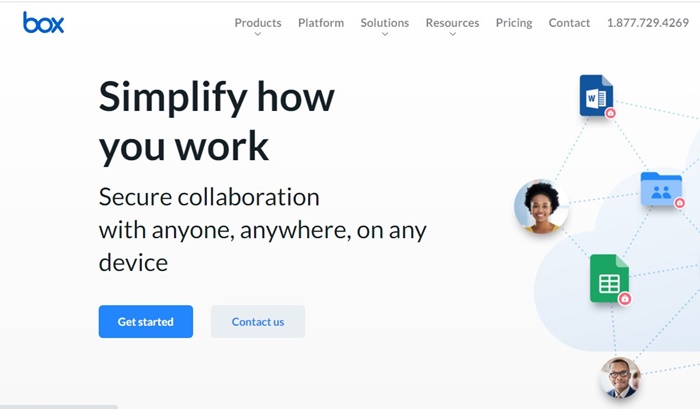This image showcases a website homepage with a clean, minimalist design. The top of the page features a thin gray border, while a thicker gray line runs horizontally from the bottom left corner for about 2 inches. The background remains predominantly white, contributing to a crisp and uncluttered appearance.

In the top left corner, the word "BOX" is displayed prominently in white, fairly large lettering. Approximately 2 inches to the right, the word "Products" is listed in black. Below "Products," a small downward arrow (greater than sign) indicates a dropdown menu. Following this, the navigation menu includes "Platforms & Solutions," "Resources," "Pricing," and "Contact." In the top right corner, the contact number 1.877.729.4269 is displayed.

To the right, a section with a faint green shading contains various elements connected by dotted lines. These include a blue WordPress icon, an African American woman's profile picture, a blue folder, another green WordPress icon, and an African American man wearing glasses.

Directly below the "BOX" logo, about an inch down, the text "Simplify how" appears in bold black letters, followed by "you work" underneath. In smaller black text, the phrase "Secure collaboration" appears, followed by "with anyone, anywhere, on any" and "device" on the next line. Below this text block are two tabs: a dark blue "Get Started" button with white text and a gray "Contact Us" button with light blue text positioned to its right.